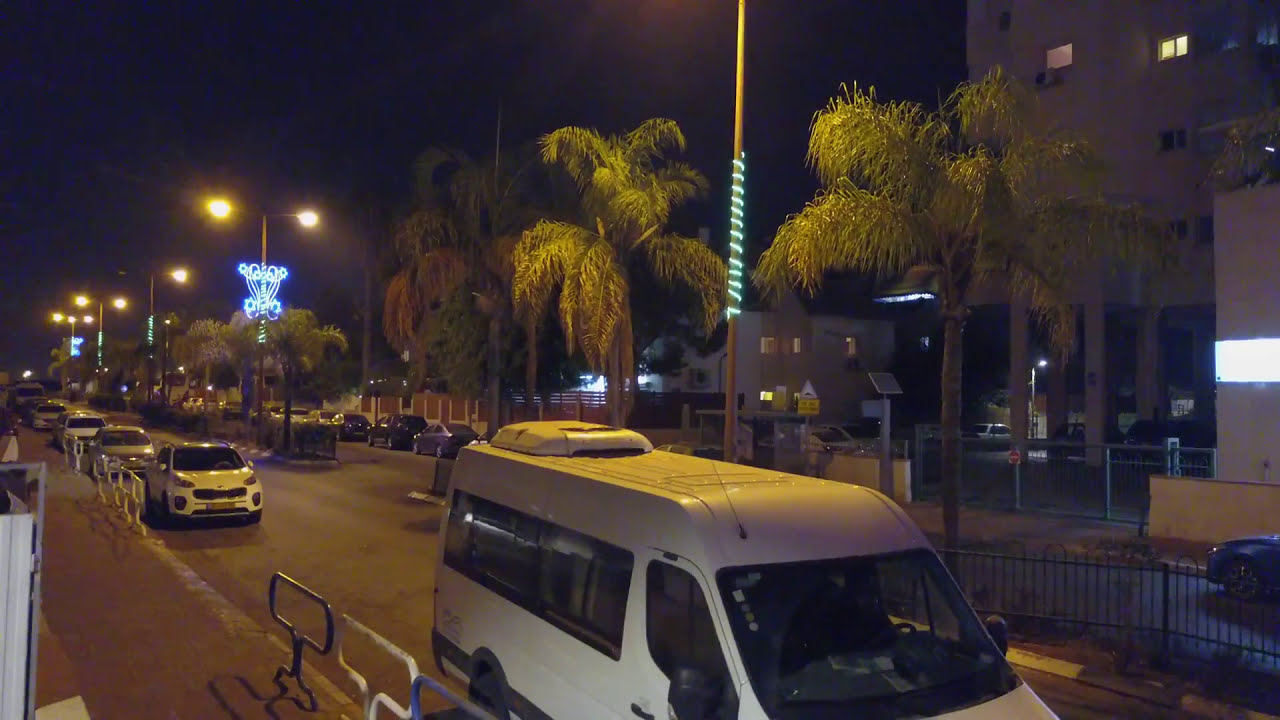The image captures a vibrant night scene in a warm climate city, characterized by a palm tree-lined center median that stretches down the street. Street lamps and string lights illuminate the area, creating a festive atmosphere. In the foreground, a white van, possibly a Sprinter or Ford Transit, is parked near a metal railing on the sidewalk. The median also features a low metal fence. The street is bordered by several vehicles parked on both sides, including a row of white cars. To the right, a building with two visible windows occupies the upper corner of the image. Decorative lights wrap around the poles, enhancing the nighttime ambiance. The street is lively with various lights, palm trees, and buildings with their lights on, suggesting a bustling urban environment.